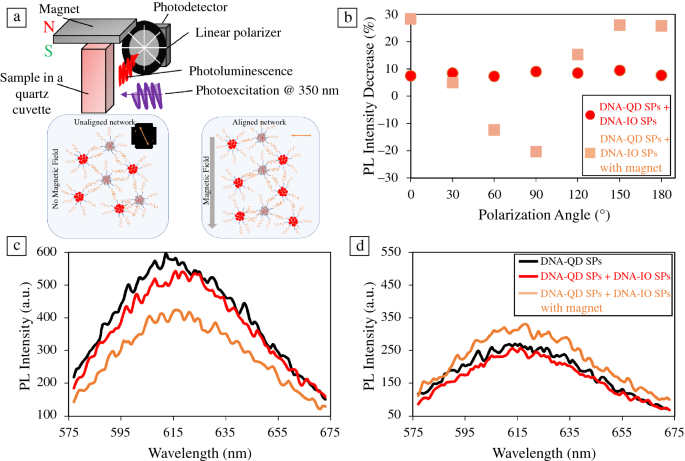The image is a detailed scientific infographic on a white background, primarily illustrating three graphs and an annotated diagram on the left. The diagram on the left features a setup where a sample is placed in a quartz cuvette and interacted with various components such as a photodetector, linear polarizer, and indicates photoluminescence and photoexcitation at 350 nanometers. This section is marked with arrows pointing out different parts like a magnet sample, with numerous red dots highlighting specific points of interest.

On the right, the top graph displays data points in the form of red dots and orange squares, where the x-axis represents the polarization angle, and the y-axis indicates the percentage decrease in PL intensity. Below this, there are two additional line graphs, each charting wavelength on the x-axis (ranging from 575 to 675 nanometers) against PL intensity (measured in arbitrary units (AUs)) on the y-axis, which spans from 100 to 600 AUs. These line graphs exhibit multiple colored lines, including orange, red, and black, demonstrating different data sets and their variations in PL intensity with respect to wavelength.